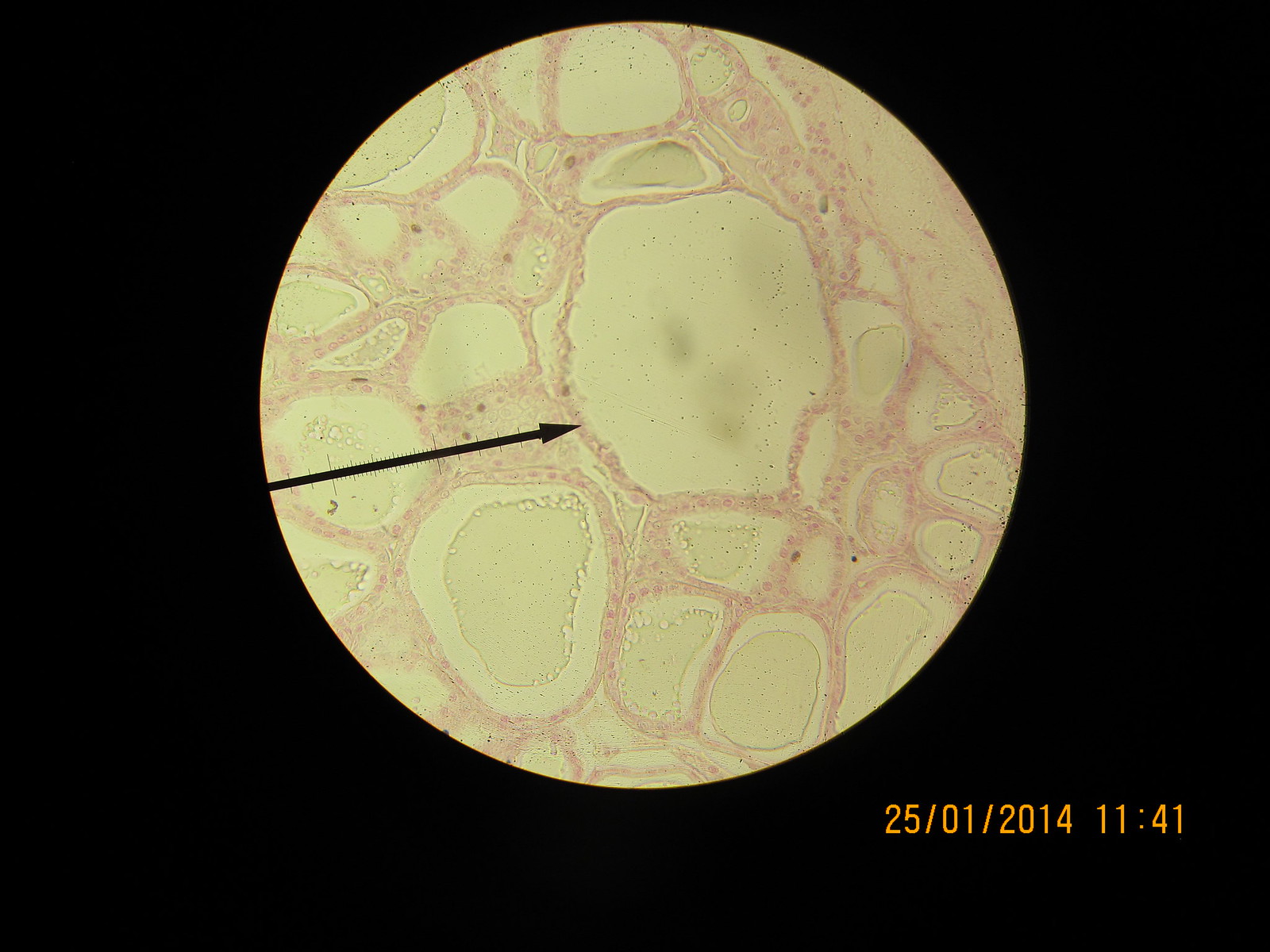The image depicts a close-up view of organic matter, possibly cell tissue or skin, captured through a microscope. The central focus of the image is a perfectly round, ivory-yellowish structure against a stark black background, as if viewed through a lens. This main structure is interspersed with various pale yellow circles, separated by pinkish membranes that have darker reddish-pink outlines. Among these circles, the largest one is marked by a black arrow pointing to an obscure dot at its edge, suggesting a point of interest that may require specialized knowledge to fully understand. The photo also includes a date and time stamp at the bottom right, reading "25-01-2014, 11:41."